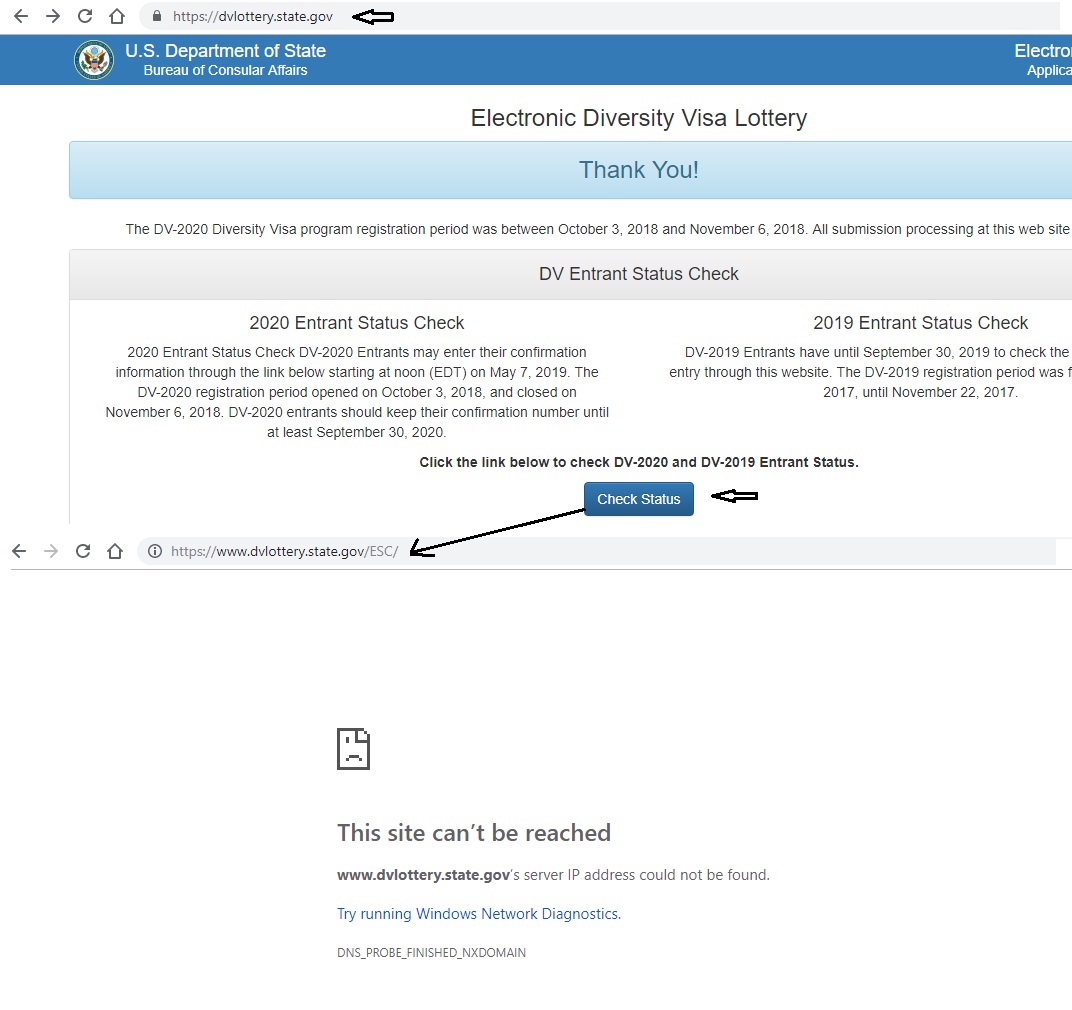The image depicts a webpage with a clean white background. At the top, there are navigation icons including left and right arrows, a refresh symbol, and a home icon. Below this, a light blue bar displays the URL "https://dvlottery.state.gov" with a prominent leftward arrow. 

A darker blue section follows, showcasing the U.S. Department of State's seal and the text "U.S. Department of State, Bureau of Consular Affairs" (correcting an initial misstatement "Consumer Affairs"). Beneath this, a white box bears the title "Electronic Diversity Visa Lottery," leading into another blue box that reads "Thank You."

The image continues with a white box indicating, “The DV-2020 Diversity Visa Program registration period was between October 3rd, 2018 and November 6th, 2018. All submissions processing at this website.” Below that, a light blue box titled "DV Entrant Status Check" appears.

In a broader white background area, more details are provided about the 2020 Entrant Status Check:
- "Entrants may enter their confirmation information through the link below starting at noon EDT on May 7th, 2019."
- "The DV-2020 registration period opened on October 3rd, 2018 and closed on November 6th, 2018."
- "DV-2020 entrants should keep their confirmation number until at least September 30th, 2020."

To the right, information regarding the 2019 Entrant Status Check is given:
- "DV-2019 entrants have until September 30th, 2019 to check their entry through the website."
- "The DV-2019 registration period was from October 18, 2017 until November 22, 2017."
- "Check the link below to check DV-2019 Entrant Status."

There is a blue box labeled "Check Status" adjacent to:
- A black arrow pointing left, next to a black arrow pointing down towards the "https://dvlottery.state.gov."

At the bottom, an icon of a sheet of paper with its top right corner bent shows a sad face, accompanied by the message "This site can’t be reached," suggesting to "try running Windows Network Diagnostics."